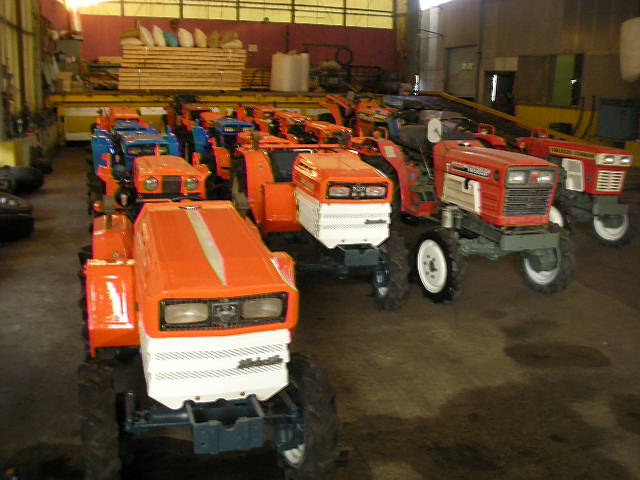The image depicts the interior of a large garage or warehouse with a cement floor and metal walls, featuring silver beams and white sides. Dominating the scene is a neatly arranged grid of at least twelve small tractors or large lawnmowers in various colors, primarily orange and red, with two blue ones included. These vehicles have black wheels with white inner rims. In the background, a red wall is partially obscured by a platform holding a stack of horizontally placed light brown lumber and a large, white circular object that appears to be plastic. On the far right side is a large gray door marked with the letter 'M' in white, accompanied by another smaller blue doorway. Additionally, bags are stacked on the lumber, and scattered oil stains are visible on the concrete floor. Tires can be seen on the left edge of the image, adding to the industrial atmosphere.